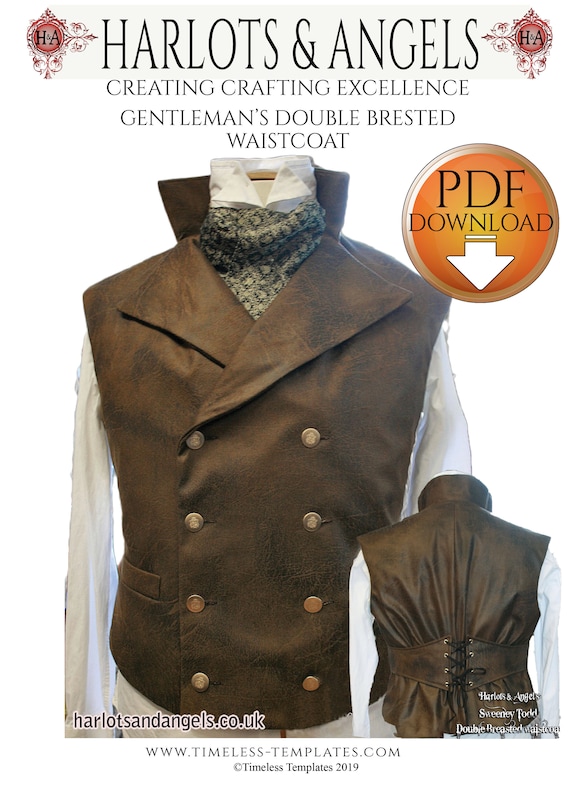This detailed advertisement for Harlots and Angels showcases their craftsmanship excellence in gentlemen's double-breasted waistcoats. Prominently featured at the top are two red circular logos, each bearing the initials “H&A” and adorned with swirling divine designs. The central text reads, "Harlots and Angels: Creating Crafting Excellence - Gentlemen's Double-Breasted Waistcoat." Below, there is a detailed picture of a brown, leather-like waistcoat displayed over a white shirt with long sleeves. The finely made waistcoat exhibits two columns of four bronze-colored buttons, each embossed with an intricate symbol. To the bottom right of the main image, a smaller view illustrates the waistcoat's back, which features a corset-like adjustable black lacing. The advertisement also includes a gradient circle transitioning from brown to tan with an orange center, indicating a PDF download option, marked by a white arrow and line above it. Key website details are present, such as "harlotsandangels.co.uk" in the lower left corner and "www.timelesstemplates.com" with a copyright symbol "Timeless Templates since 2019" underneath the image, though some smaller text on the lower right remains illegible.